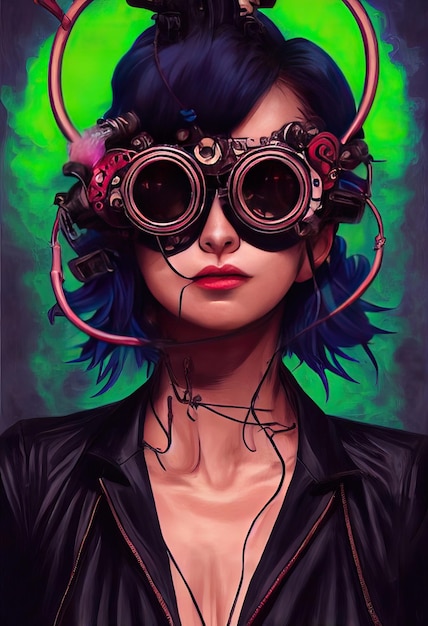The image is a detailed painting or AI-generated art that evokes a comic book aesthetic, depicting a futuristic, steampunk-style woman. The centerpiece of the art is a woman wearing large, round, chrome-steampunk goggles adorned with numerous wires. One prominent wire extends from her goggles into her mouth, loops around her neck, and cascades down her chest. Thick pink cords dangle from the sides of the goggles, disappearing into an indistinct device on her head, which is partially visible. Her hair is a striking dark blue, styled in a low updo, paired with bold red lipstick. She is dressed in a sleek black leather jacket, exuding a professional and content demeanor. The background contrasts sharply with the main figure, featuring a black backdrop with swirls of eerie green fog. The entire composition radiates a vivid, futuristic vibe, and utilizes a palette of blues, neon greens, blacks, and grays.